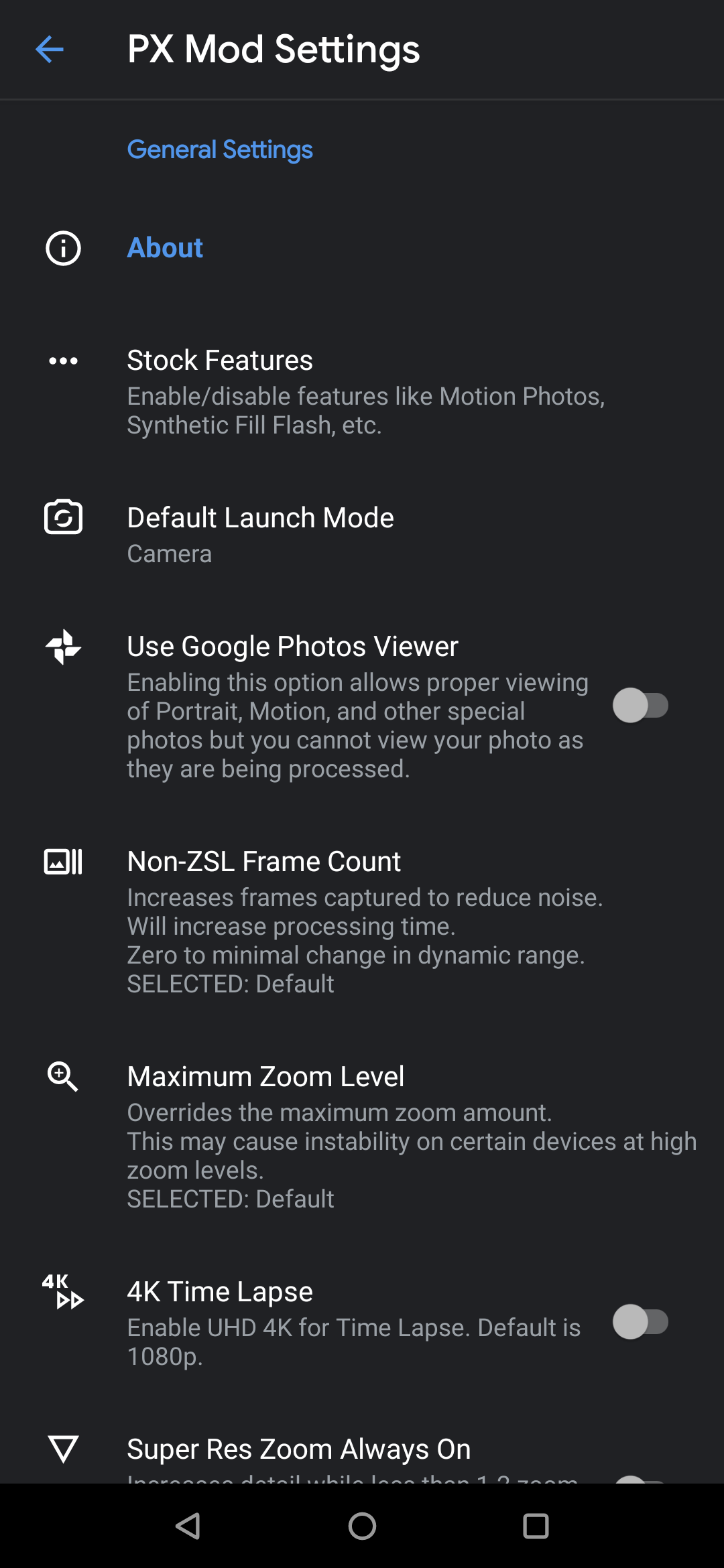**Detailed Caption:**

The image showcases a user interface screen set against a black background. At the very top of the screen, there is a blue arrow pointing to the left, followed by the text "PX Mod Settings" written in white. Below this text is a thin horizontal line that spans the width of the screen. 

Underneath this line, the heading "General Settings" is written in blue. Close to this heading, there is a white circle featuring a capital letter "I" in its center. To the right of this circle, the word "About" is written in blue text.

Further down, there are three horizontal white lines which segment this section from the subsequent text. All the following content is written in white. The next section is labeled "Stock Features", which includes a description that reads: "Enable, Disable features like Motion Photos, Synthetic Fill, Flash, etc."

Beneath this description, there is a camera icon followed by the text "Default Launch Mode: Camera". Then, a small whirly wheel icon appears before the text "Use Google Photos Viewer". A detailed note beneath this field states: "Enabling this option allows proper viewing of portrait, motion, and other special photos, but you cannot view your photo as they are being processed." An adjacent toggle switch, positioned to the right, is currently in the off position.

Next, a square icon with two intersecting arrows and two horizontal lines is labeled "Non-ZSL Frame Count", accompanied by the information: "Increases frames captured to reduce noise. Will increase processing time. Zero to minimal change in dynamic range." This option is marked as the default setting.

Following this, a magnifying glass icon appears next to the text "Maximum Zoom Level", with a note explaining: "Overrides the maximum zoom amount. This may cause instability on certain devices at high zoom levels." This setting is also selected as the default.

A "4K" icon with two arrows pointing to the right precedes the text "4K Time Lapse", described as: "Enable UHD 4K for time lapse. Default is 1080p." This feature includes a toggle switch which is currently turned off.

Below, there is an upside-down triangle followed by the text "Super Res Zoom Always On". Slightly obscured text beneath this is partially visible but cut off.

At the very bottom of the screen, there are three icons: an arrow pointing left, a circle, and a square, representing common navigation buttons.

This detailed caption provides a comprehensive description of the image's contents and the various settings available on the interface.